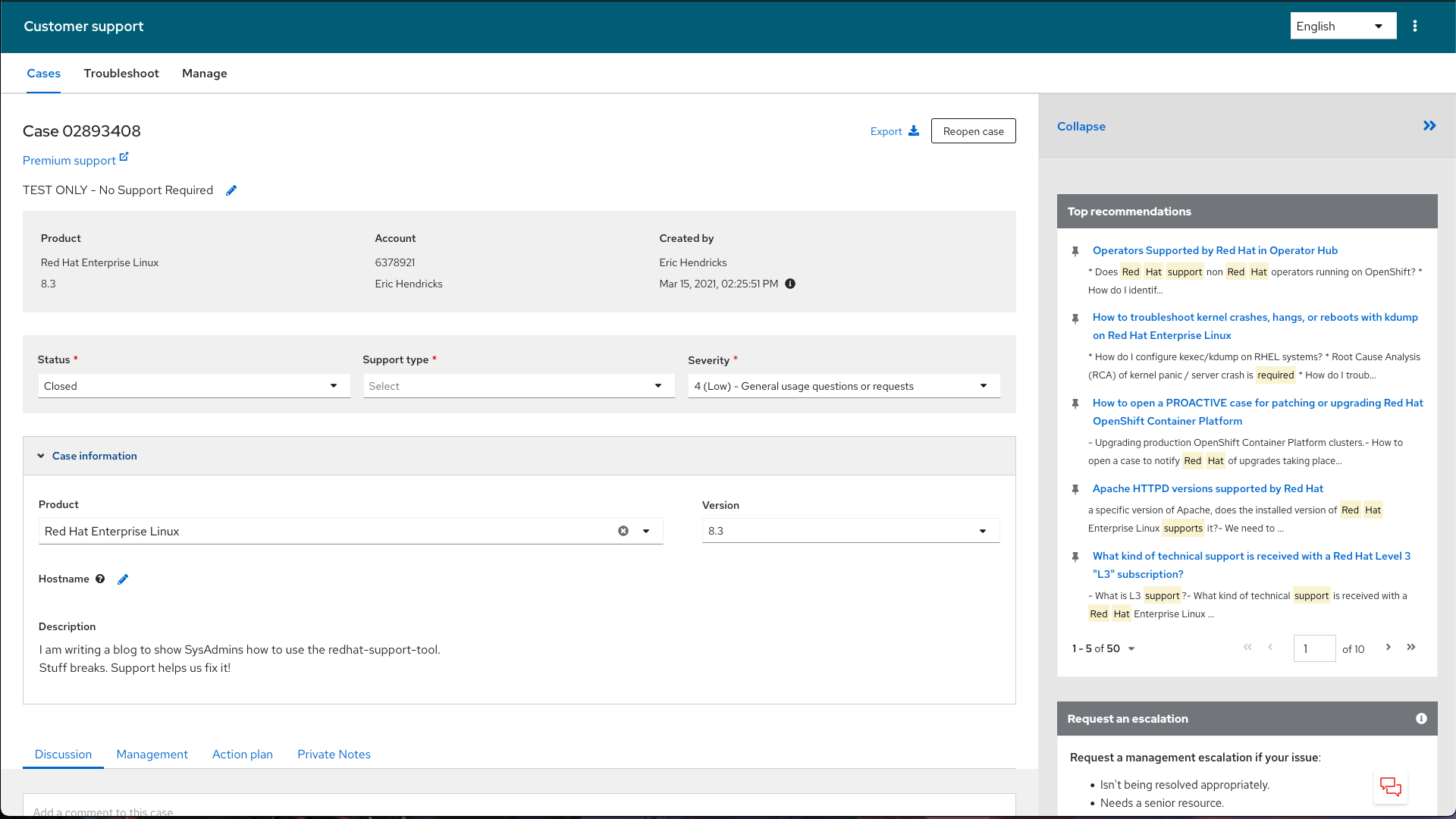The image depicts a customer support interface related to consumer support. Central to the image is a support ticket, identifiable by a unique case number that has been created. Although the text on the ticket is very small and illegible, you can make out several gray fields that likely contain pertinent details. In the top left corner, black text is seen, potentially indicating metadata or labels for the ticket. 

The top right section of the interface features a recommendation form, possibly generated by a chatbot, with several items highlighted in yellow for emphasis. A teal banner spans across the top, prominently displaying "Customer Support Ticket." Additionally, a blue-colored "Premium Support" link is visible, suggesting an option for enhanced customer service.